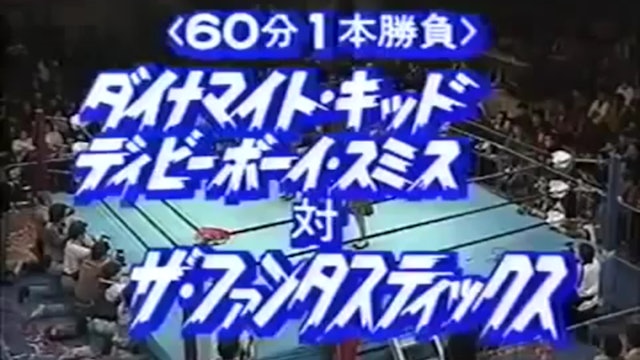The image depicts a boxing ring or wrestling ring set in a dark arena, surrounded by a large audience. The scene is dominated by a light blue floor of the ring, bordered by ropes on all sides. The audience, comprising people sitting, standing, and kneeling at the ring's edge, includes photographers capturing the event. The ring's central detail is partially obscured by large white text and symbols in a non-English, possibly Asian, language. This text is highlighted with a bright blue background, stretching from the top to the bottom of the photo. Among the text, the very top reads "6-0," followed by a sequence of characters including the number "1" and other symbols. Glimpses through the text reveal only a leg, suggesting the presence of a person inside the ring, likely a participant in the event.